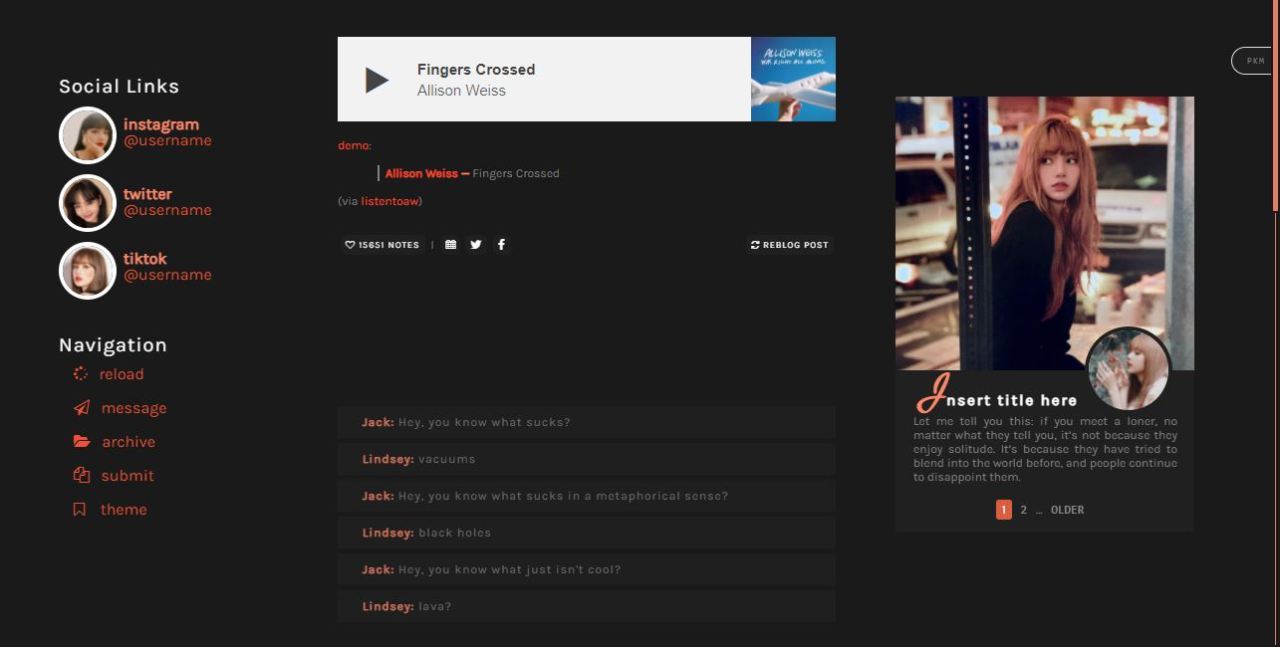**Detailed Caption:**

The image depicts a web page template that is in the process of being customized. On the left side, there is a section titled "Social Links" featuring three circular placeholder images of women, which are likely intended for the user's own photographs. Each image is labeled with a social media platform followed by "@username": Instagram, Twitter, and TikTok, indicating customizable links for the user's social profiles.

Below the "Social Links" section is a "Navigation" menu containing options such as Reload, Message, Archive, Submit, and Theme. These likely offer functionality to navigate and personalize the web page.

At the top of the page, a white bar displays the text "Fingers Crossed" followed by "Alison Weiss" and a play button, suggesting a musical feature—perhaps a song by an artist named Alison Weiss. Directly below this is a partially readable text, which appears to say "Demo" and repeats "Alison Weiss, Fingers Crossed via [unreadable text]." Accompanying this text are icons for Twitter, Facebook, and another social media platform, indicating sharing options.

Further down, there's a conversation displayed in a chat format between two individuals named Jack and Lindsay. Their humorous exchange includes:
- Jack: "Hey, you know what sucks?"
- Lindsay: "Vacuums."
- Jack: "Hey, you know what sucks in a metaphorical sense?"
- Lindsay: "Black holes."
- Jack: "Hey, you know what just isn’t cool?"
- Lindsay: "Lava."

A profile picture of a woman with long red hair appears next, taken in what looks like a garage. She's turned toward the camera, but her gaze is directed to the far left. 

Below this profile picture, the text "Insert Title Here" indicates another customizable placeholder, with a personal quote beneath it:
"Let me tell you this, if you meet a loner, no matter what they tell you, it's not because they enjoy solitude, it's because they've tried to blend into the world before and people continue to disappoint them."

At the bottom, a navigation element lists "1" (which is highlighted), "2," and "Older," suggesting a historical timeline of posts that can be browsed.

The overall layout and remaining placeholders suggest that the template is designed for a personal or blog web page that remains to be fully personalized.Considering the lack of specific branding and the layout's features, it might be a common web page template that the viewer does not recognize.